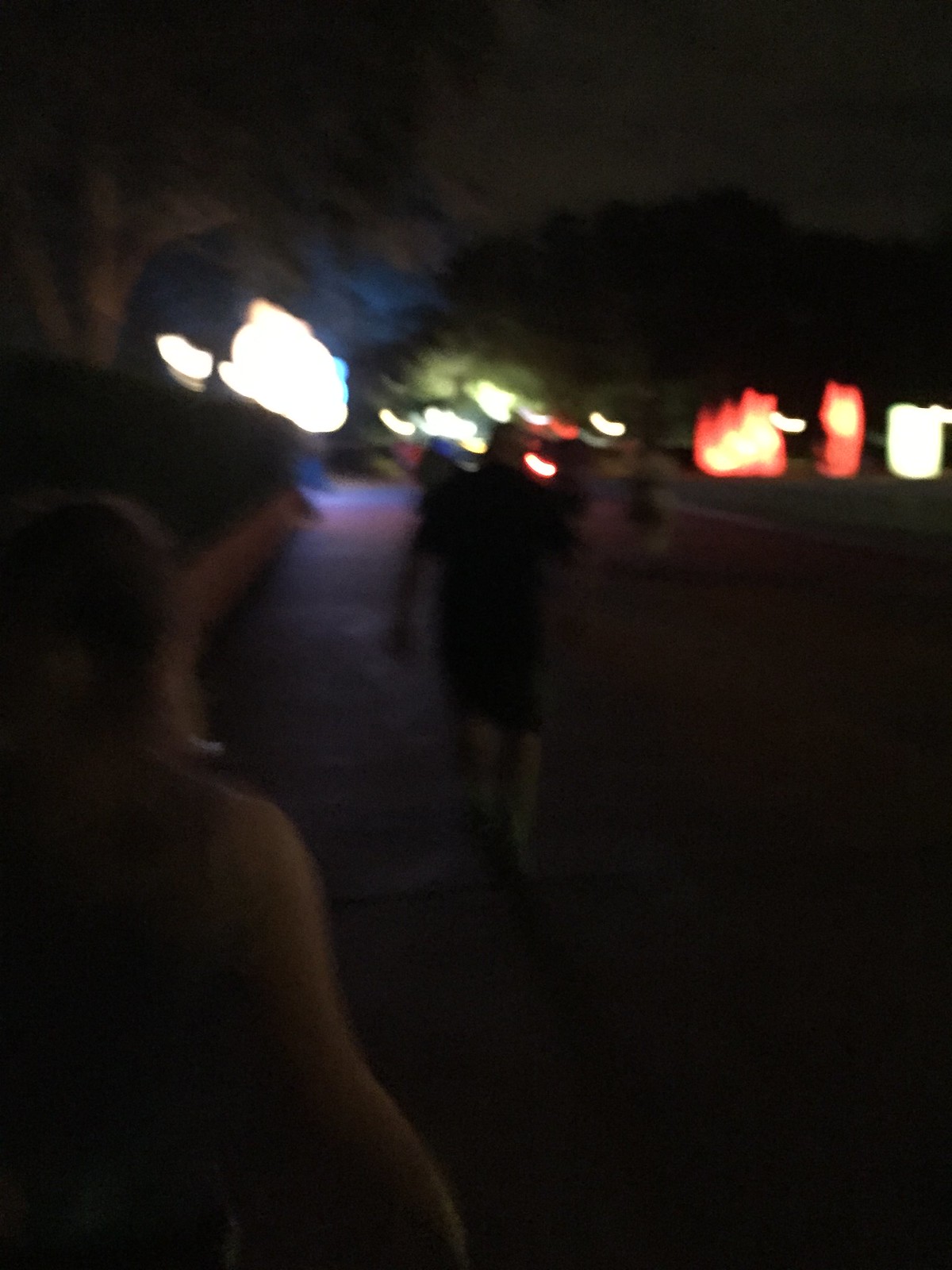In this blurry, nighttime photo, a man with a shaved head is seen walking away down the middle of a sidewalk, framed by a black t-shirt and black shorts, his right arm raised and left arm resting by his side. His white skin stands in contrast to the dark, fuzzy ambiance around him. To the left in the foreground, a younger woman with long, brown hair, draped in a sleeveless purple shirt, is visible. They appear to be near a small concrete wall that is lined with bushes and trees. Off in the distance, blurry lights illuminate the scene slightly, while a dark sky and an indistinct tree line loom in the background. On the right, vague red blurs and other indistinct figures walking down the road add to the grainy, low-quality texture of the photograph.